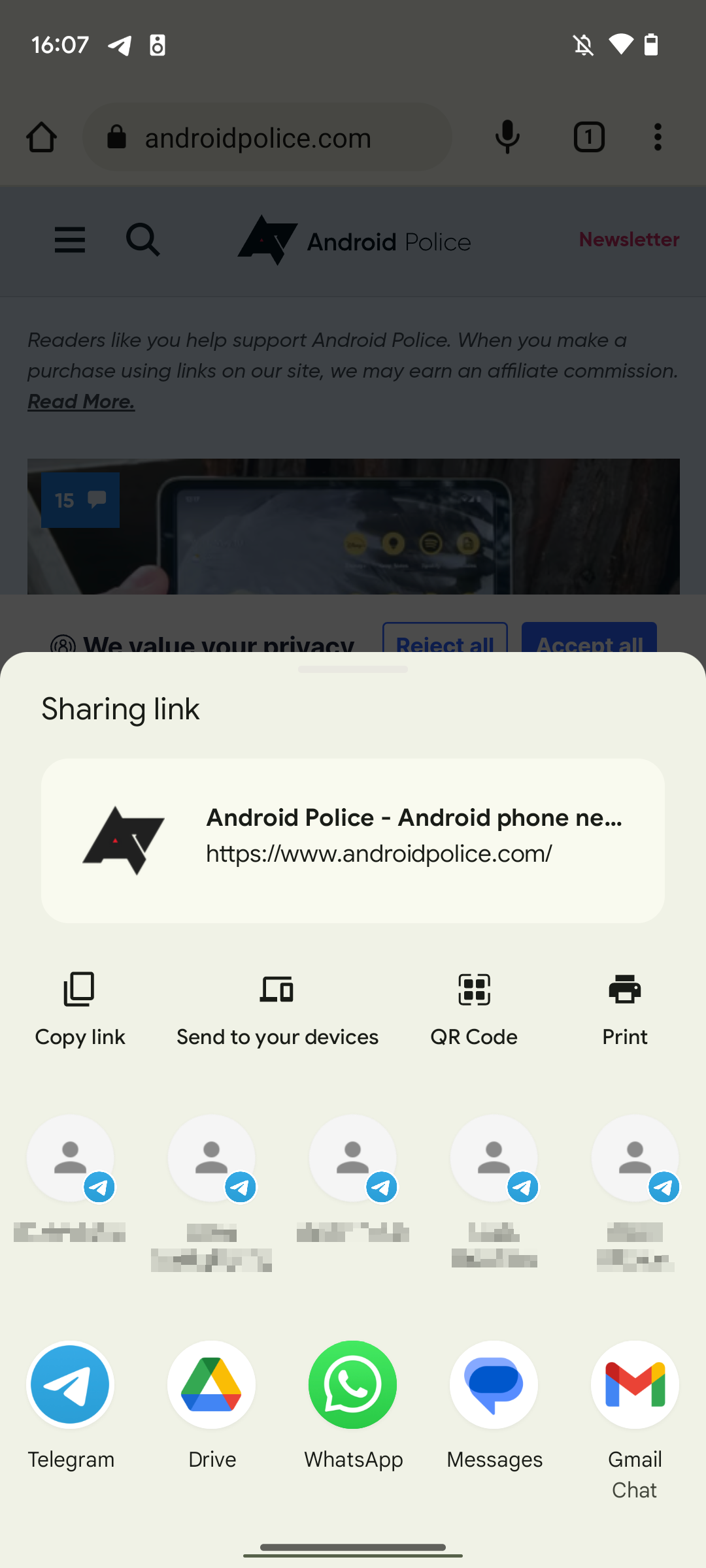This image showcases a screenshot of a mobile device's screen, predominantly displaying a sharing interface for a web link. The central focus of the image is an overlay in the bottom half, titled "Sharing link," with the URL pointing to www.androidpolice.com. Immediately beneath this title, the interface offers several actions: to copy the link, send it to the user's device, generate a QR code, or print it. 

Below these options are choices to share the link with contacts, whose details are intentionally blurred out for privacy. Further down, more app-specific sharing options are available, including Telegram, Google Drive, WhatsApp, Android Messages, and Gmail Chat.

The upper half of the image shows a partial view of the web page from Android Police, with the URL visible in the navigation bar. At the very top of the screenshot, the status bar displays essential information about the device: the current time is 16:07, accompanied by icons for a paper airplane (likely denoting a sent message), speaker, a muted symbol, WiFi connectivity, and the battery level.